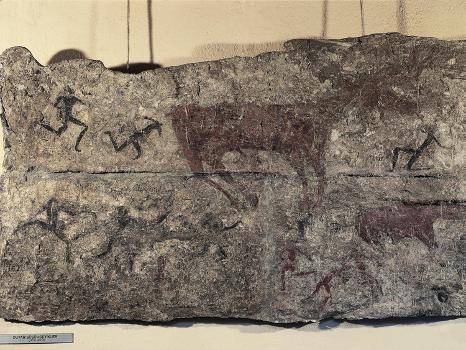In this detailed, color photograph, we see a close-up of an ancient, rectangular slab of stone resting on a white base, set against an off-white wall. To the bottom left-hand corner, a small, gray sign with black letters provides information about the artifact, though it's difficult to read due to its tiny, blurry text, possibly not in English. This historic artifact appears to be from a museum or art gallery, showcasing a profound blend of art and history.

The stone, likely hundreds to thousands of years old, features carved markings illustrating primitive scenes. Predominantly using neutral colors—gray stone, with dark black and brown carvings accented by flakes of white—the carvings depict several stick-figure-like human figures engaged in various activities. There are tall, black figures in motion, resembling ancient cave paintings. One area of the stone illustrates two men running or chasing a large animal, which appears to be a bull or cow, etched in a dark red hue. In this scene, a stick figure of a man seems to be falling backward, with one knee on the ground and the other leg bent, possibly indicating some dynamic storytelling about life and death. 

Overall, the ancient carvings on this piece of stone provide a fascinating glimpse into early human communication and artistic expression.